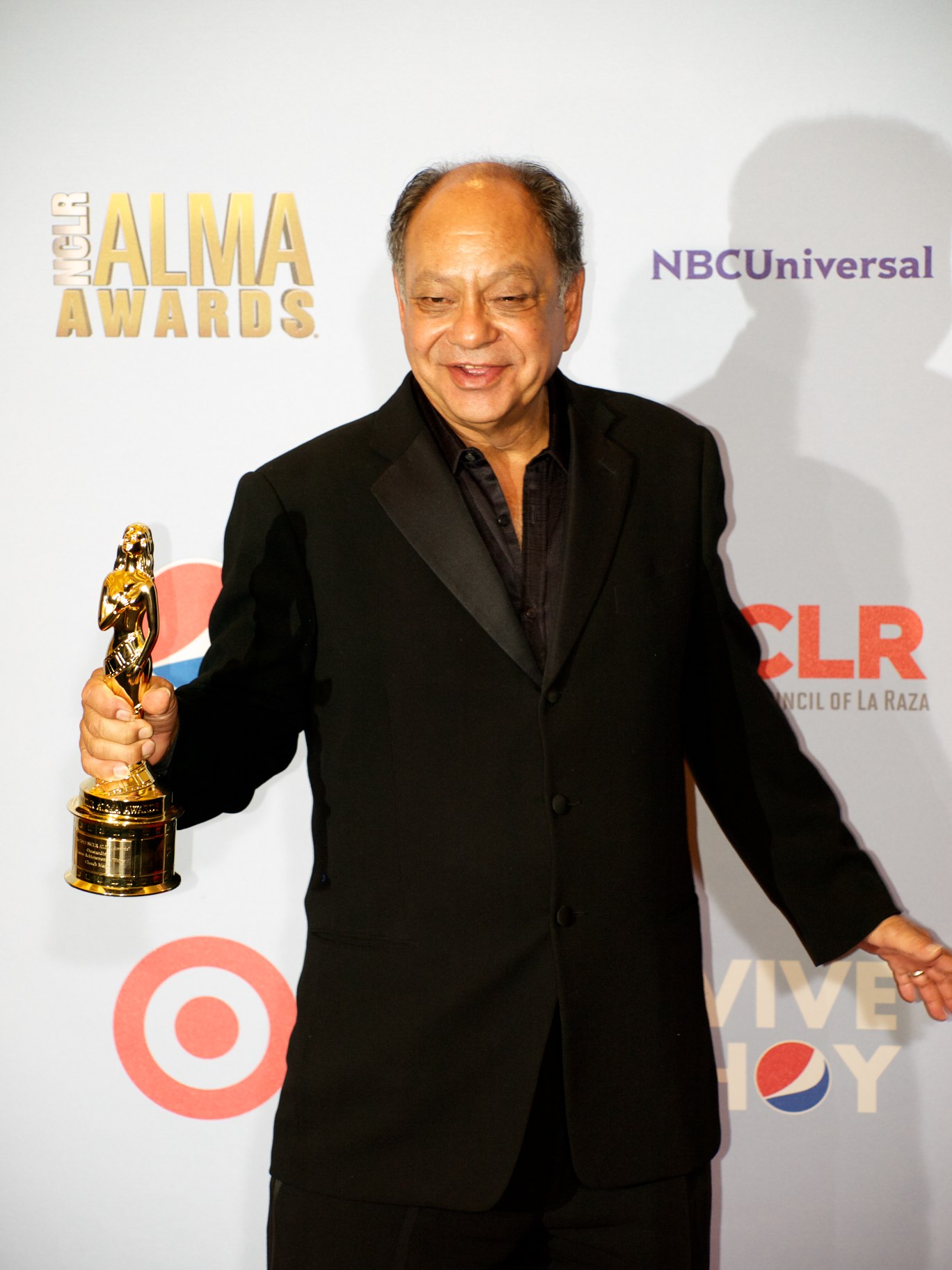This image captures an older Latino man, possibly in his 60s or 70s, standing centrally at the ALMA Awards event. He is dressed in a black ensemble, consisting of a long, somewhat ill-fitting black suit jacket, black pants, and an unbuttoned black dress shirt underneath. The man, with tanned skin, has a horseshoe hairdo with gray hair on the sides and is balding on top. His eyes show signs of age with squinting and noticeable bags. He appears joyful, smiling broadly as he holds a golden trophy in the shape of a woman with a gold base.

Behind him, a large banner displays various logos and text, emphasizing the prestigious nature of the event. The banner prominently features the text "NCLR ALMA Awards" in yellow on the upper left, "NBCUniversal" on the upper right in purple, along with the logos of Pepsi in blue and Target in red. The backdrop conveys a celebratory atmosphere, reinforcing the significance of the award in his hand.